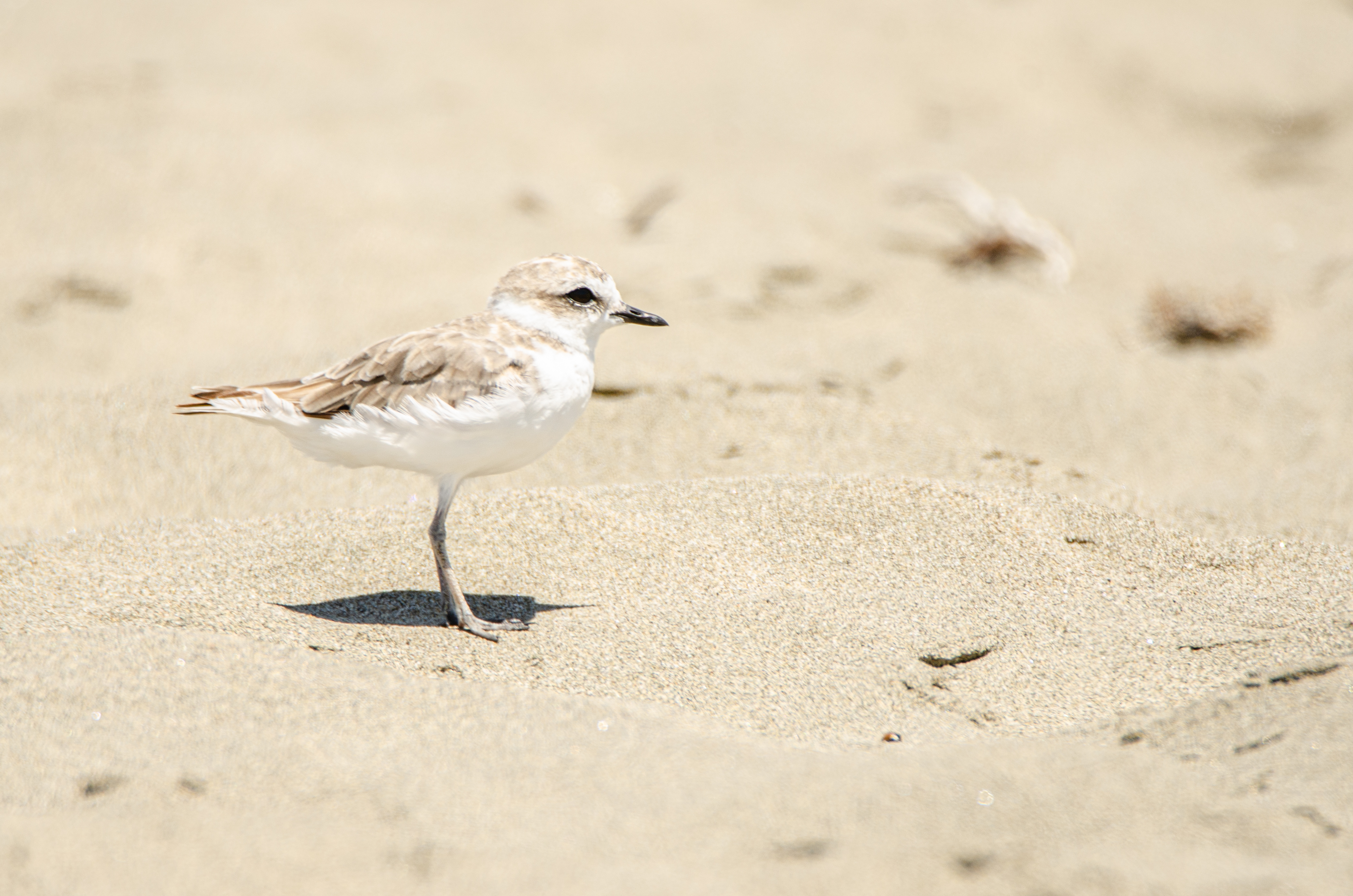The image captures a close-up shot of a small bird standing on a patch of sand. The bird, which may be a piping plover, prominently features white feathers on its belly and a ring of white around its neck, while the rest of its plumage is a mix of light brown and gray. Its head is turned to the right from the viewer's perspective, revealing one black eye and a black beak. The bird's right leg is visible with a transition from white at the top to light brown towards the bottom. Positioned on the left side of the image, the bird casts a shadow directly below, suggesting the photo was taken around midday with overhead lighting. The sandy background is featureless, save for a couple of indistinct, blurry objects in the distance.